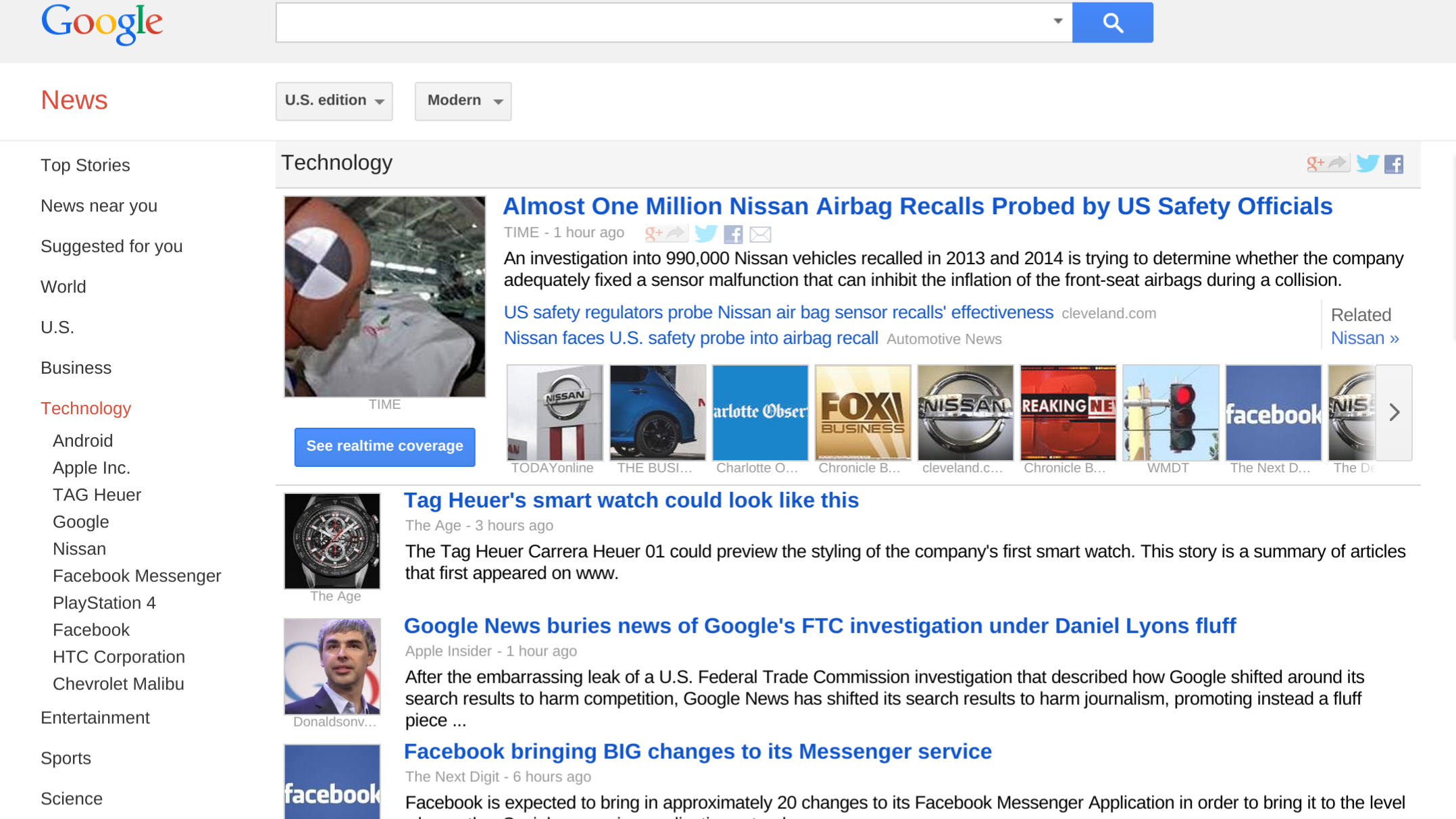Screenshot of the Google News page displaying various sections and articles.

In the center of the page, there is a prominent white search bar, accompanied by a blue button with a magnifying glass icon on the right. The "News" section is highlighted in red at the top.

On the left side of the page, the sections listed include:
- Top Stories
- News Near You
- Suggested For You
- World
- U.S.
- Business
- Technology (highlighted in red)
- Android
- Apple
- Tag Heuer
- Google
- Nissan
- Facebook Messenger
- PlayStation
- Facebook
- HTC
- Chevrolet Malibu

Further down, additional sections listed are:
- Entertainment
- Sports
- Science

On the right side of the page, it is labeled as "U.S. Edition" and the theme is denoted as "Modern."

Highlighted articles in the "Technology" section include:
1. "Almost 1 million Nissan airbags recalled, probed by U.S. safety officials" with a corresponding image of an airbag.
2. "Tag Heuer Smart Watch could look like this" with an accompanying image of a watch.
3. "Google News buries news of Google's FTC investigation" by Daniel Lyon, with a picture of a person next to it.

The page layout presents a clean and organized overview of current news and sections tailored for the user.